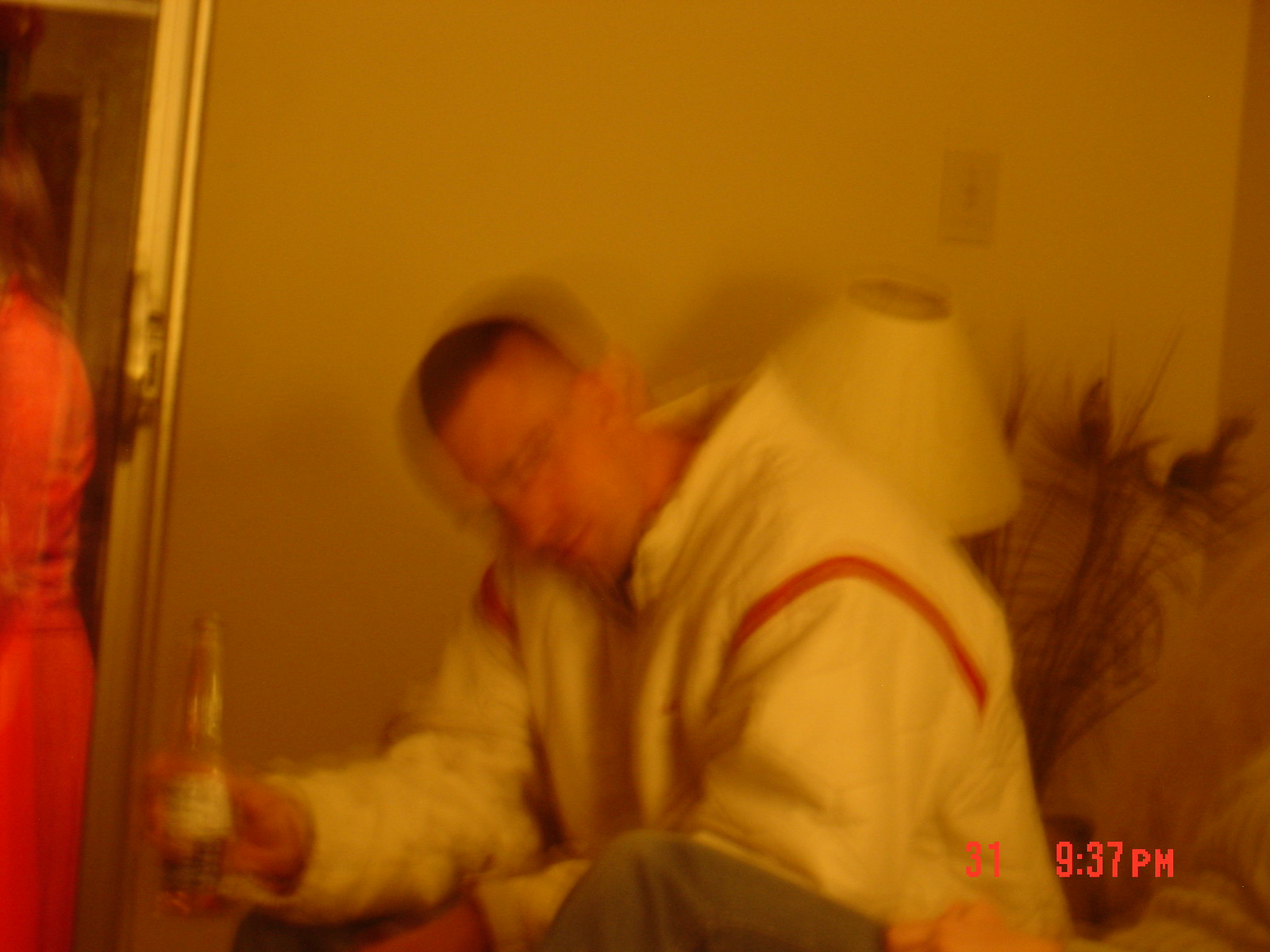The image is a blurred photograph, likely captured with a regular camera in a light gray painted room. At the center of the frame is a man with light skin and short dark hair, wearing a white jacket with bright red piping. He appears to be in mid-movement, causing the blur, and is holding a clear glass bottle with a white and gold label in his right hand. There is a timestamp at the bottom right corner in red digital text reading "31 9:37 p.m."

To the left of the man, a metallic silver doorway is partially visible, showing the back of a person with shoulder-length white-brown hair, wearing a bright orange dress. This individual stands partially cropped out of the frame. Behind the man, there is a white, askew lampshade and a plastic-framed light switch mounted on the wall. Below the lampshade and light switch, decorative light brown plants, or possibly feathers, are sticking out. The overall setting suggests an indoor environment, possibly a house.